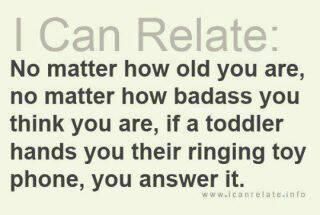The image features a simple, text-based design on a cream-colored background. At the top, in large, thin, gray text, it reads "I Can Relate," with each word capitalized. Directly below this, in bold black text spanning across approximately five lines, is the phrase: "No matter how old you are, no matter how badass you think you are, if a toddler hands you the ringing toy phone, you're gonna answer it." At the bottom, in a smaller, faded gray font, is the URL "www.icanrelate.info." The entire image maintains a clean and minimalist aesthetic with an Arial typeface, and emphasizes the humorous universal truth conveyed in the text.